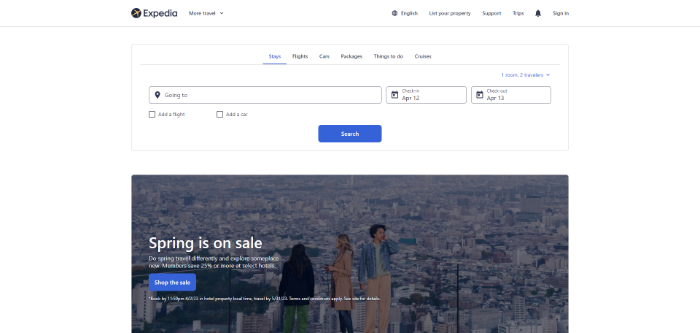The image depicts a screenshot of the Expedia website displayed against a white background. At the very top, the Expedia logo is prominently featured with a capital "E" in larger text. Next to the logo, there is a drop-down menu with the label "More Travel," indicated by a down arrow. To the right of this, the text "English" appears, accompanied by four tags that are blurred and difficult to read.

Moving further right, there is a small bell icon, which likely serves as a notification symbol. Below this navigation bar, a white square encapsulates various elements against the white background. Within this square, the first section features blue text with an underline, but the text is unreadable due to blurriness.

Centered in the square is a search bar labeled "Going to," suggesting the user can enter a destination. Below this, there are options with small squares to add a car rental or a flight. The check-in and check-out dates are listed as April 12th and April 13th, respectively. Finally, a search button is present.

At the bottom of the image, there is a graphic of a cityscape with a caption indicating a special offer: "Spring is on Sale."